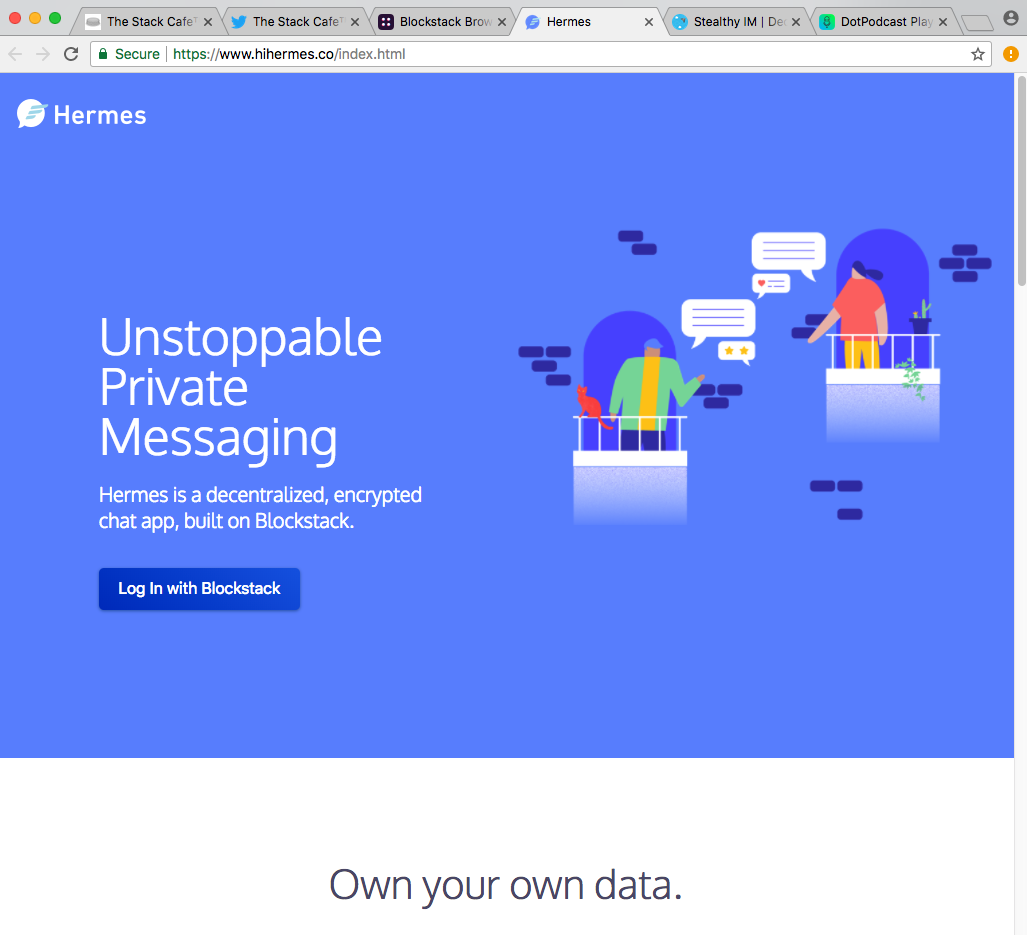The image is a detailed screenshot of the Apple Safari web browser displaying the Hermes website. The browser features the classic stoplight buttons in the upper left-hand corner: a red dot, a yellow dot, and a green dot. There are six open tabs as follows, from left to right: Stack Café, Stack Café with a Twitter icon, BlockStackBRWOW, Hermes (the current tab), Stealthy IM with a logo, and a .podcast player with a bright green icon featuring a thumbtack outline in black.

In the upper right-hand corner of the browser, a grey profile icon featuring a light grey person is visible against a dark grey background. The navigation controls below the icon include left and right back and forward buttons, and a refresh button. The secure connection is indicated by a padlock next to the website URL, https://www.hihermes.co.html. Toward the far right of the navigation bar, there is an empty bookmark star and an orange button with a white exclamation mark.

The current tab displays the Hermes website. The upper left-hand corner features the Hermes logo, a feather inside a white circle, accompanied by the text "Hermes" and "Unstoppable Private Messaging" in white. Hermes is described as a decentralized encrypted chat app built on Blockstack. Below this text is a dark blue button labeled "Login with Blockstack."

The website's background is a lighter blue color, and the right-hand side of the page depicts two people conversing from adjacent balconies. The lower balcony has a man in a green sweater over a yellow t-shirt and blue pants, standing beside a red cat. He is engaging in a conversation with a woman on an upper balcony, dressed in a red t-shirt and yellow pants, with plants adorning her balcony. Both characters are represented with speech bubbles, indicating an active conversation.